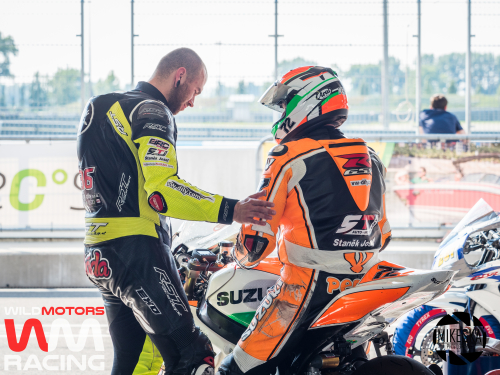In a smaller square photograph taken inside a bright showroom with large blurred windows revealing trees outside, two men dressed in eye-catching motocross gear are showcased. The man on the left, a white individual with a shaved buzzcut, stubbly beard, and gauges in his ears, dons a black and yellow racing suit adorned with numerous logos. He is in profile, facing right, and appears to have a distinct hump under his shirt, possibly protective gear. His right arm rests on the left shoulder of another man positioned at the center of the photo, sitting atop a sleek white Suzuki motorcycle with green and black accents. The rider, clad in a striking green, white, and black suit, wears a matching helmet, obscuring his face. Below them, in the lower left corner, the text "Wild Motors Racing" is clearly visible, emphasized in bold red and white lettering next to a "WM" logo. Outside, hints of a dirt track and fences can be seen in the vibrant outdoor scene bathed in daylight.